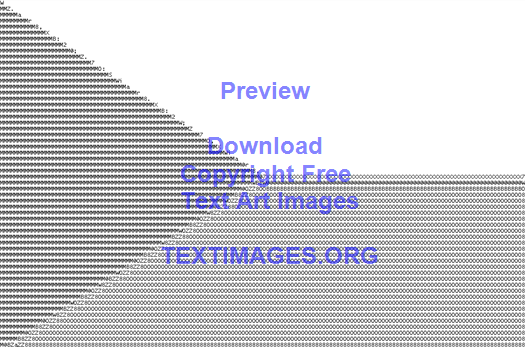The image is a black-and-white typographic design in landscape orientation, characterized by a triangular area on the left composed of an array of W's and M's, and a rectangular shape at the bottom emanating from the triangle, both made up of light gray computer characters. The upper and right-hand sections of the image are blank, creating a stark contrast. Centered in the white space at the top, there is blue text reading "Preview" and "Download". Overlapping the gray-text areas of the triangle and rectangle, more blue text states "Copy Free" followed by "TextArt Images" and the URL "TextImages.org". The detailed combination of a geometric design and text highlights the graphic style of typography and text art.